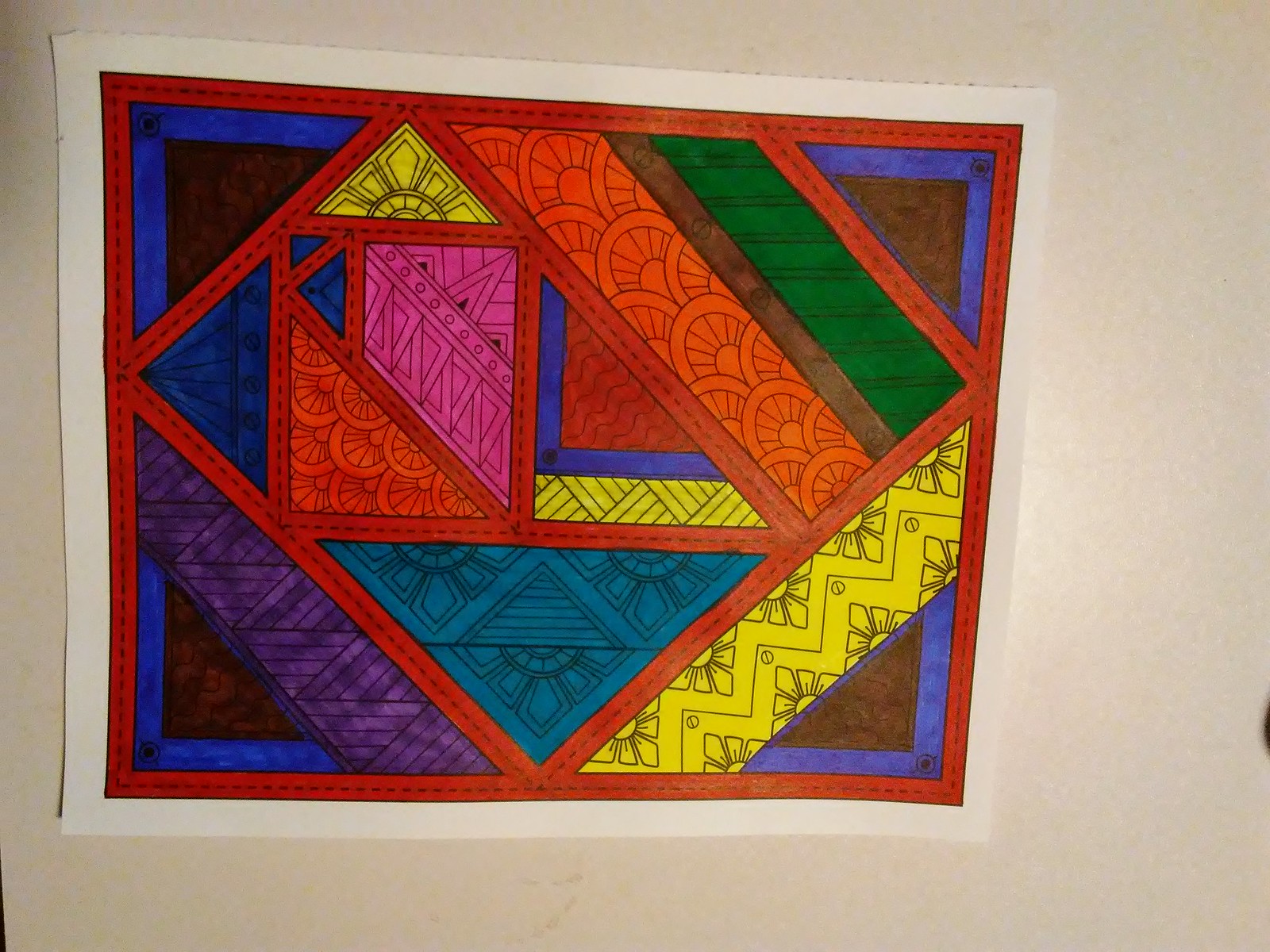A vibrant and brightly colored drawing set against a drab, off-colored wall captures immediate attention. The artwork is framed by an off-white border, accentuating the contrast between the vivid interior and the subdued surroundings. Within this frame, an orangish-red border further defines the piece and delineates the geometric sections. The design consists of an eclectic mix of geometric blocks and triangles, featuring an array of lively colors including pink, orange, yellow, green, blue, turquoise, purple, and brown. The internal lines of orangish-red divide the artwork into various segments. Each segment is uniquely filled with patterns—some showcasing flowers, others adorned with more triangles, and many featuring vibrant stripes. The geometric shapes, characterized by sharp angles and randomly arranged, create a dynamic and visually stimulating composition.